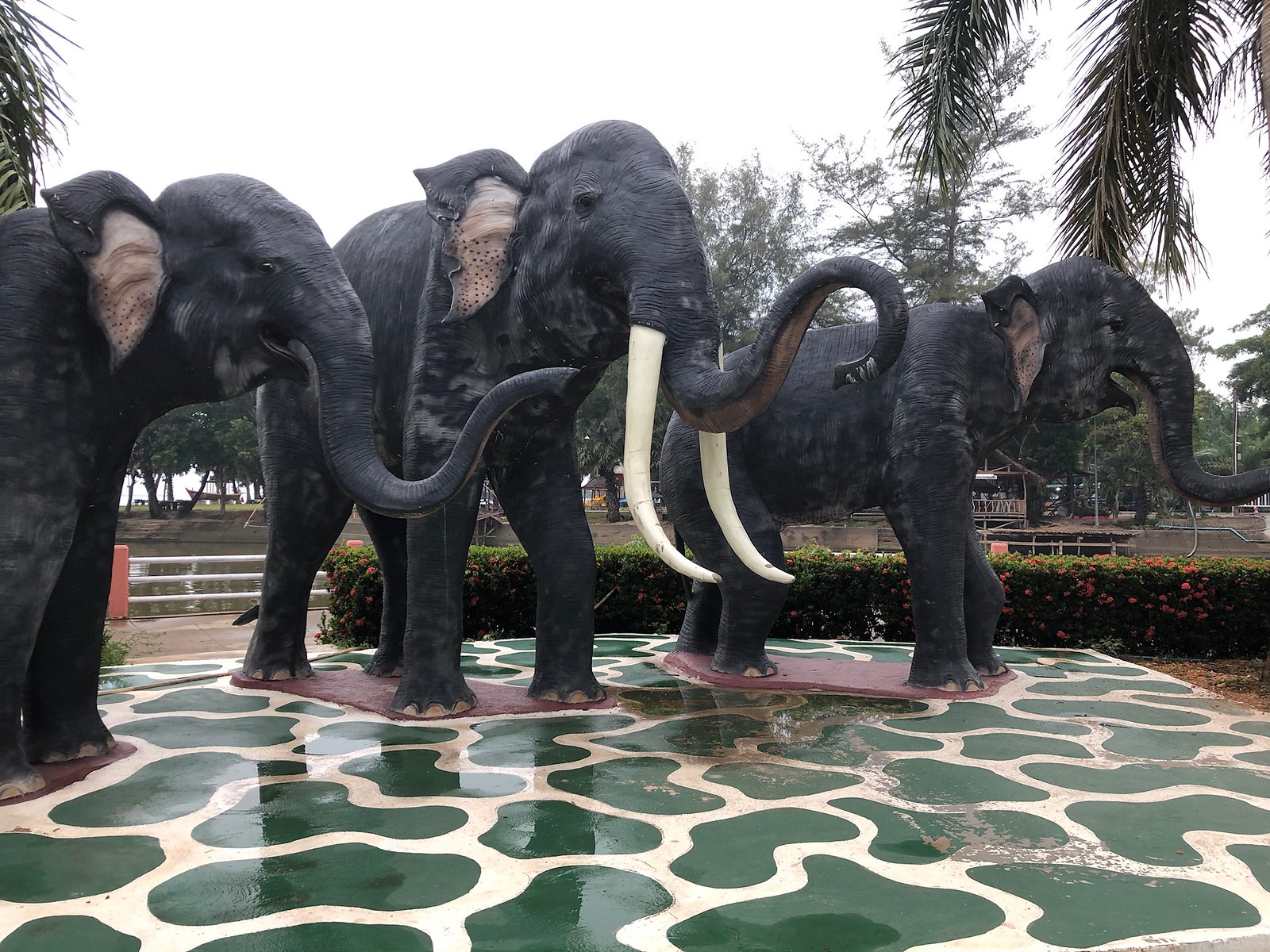In this daytime photograph taken from waist height, we see three life-size elephant statues positioned in an outdoor park setting. The statues are deep dark gray, almost black, deviating from the typical color one would expect. The elephants are arranged in a row, all facing towards the east. The middle elephant stands out with its prominent white tusks and a curled trunk, while the other two, appearing younger and without tusks, have their trunks sticking out to the sides. All three statues have their ears lifted slightly, exposing the pale, fleshy interior. The statues are placed on individual dark brown stone stands atop a geometric green and white tile patio, which intriguingly features a pattern reminiscent of a giraffe's spots. The backdrop is filled with trees, shrubbery, and possibly some seating benches, giving a sense of a park-like or zoo setting. The sky is overcast, adding to the unique ambiance of the scene.